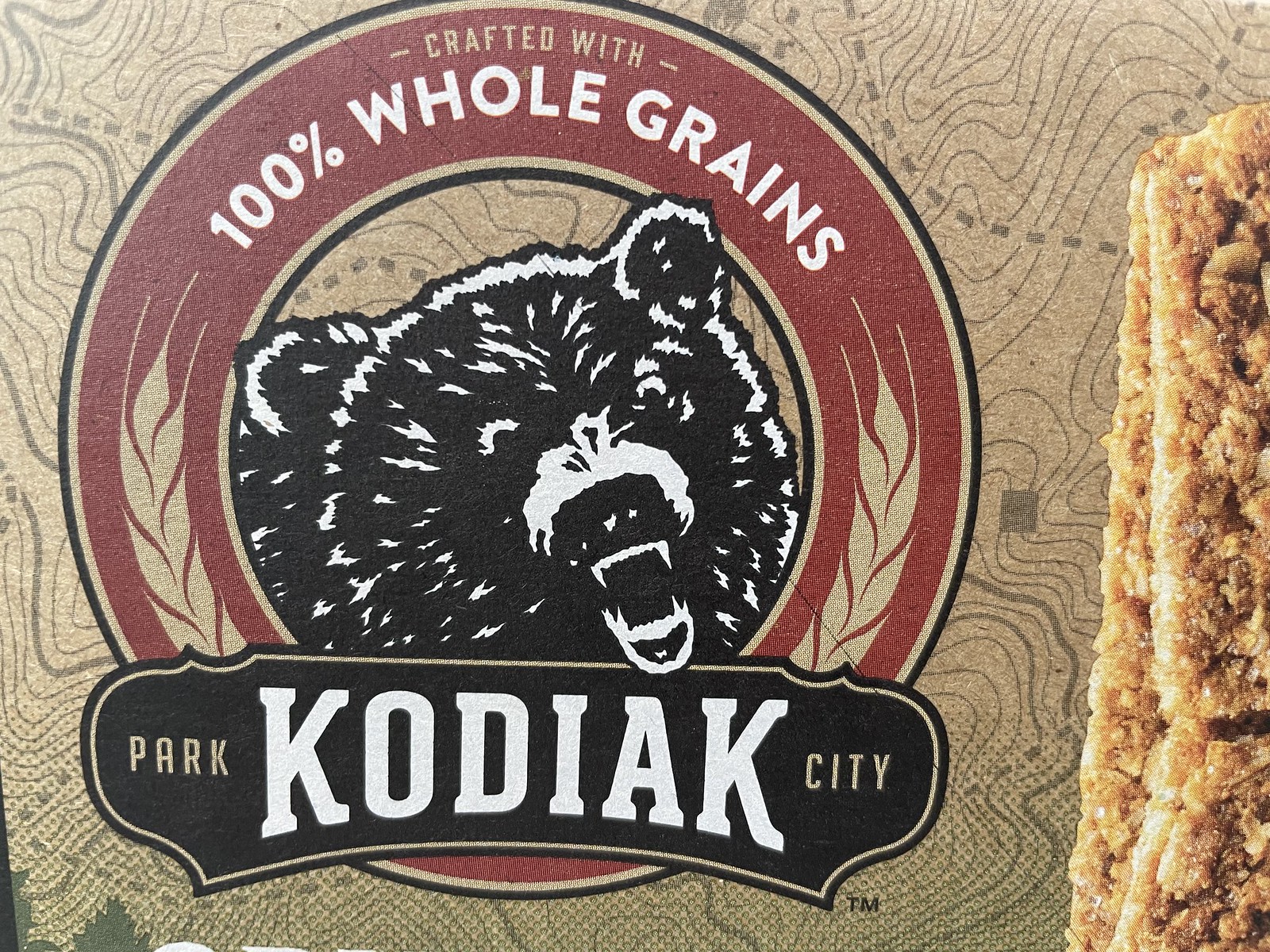This is a detailed image of the front packaging of a brand known for granola bars. The focal point is a prominent, dark red circular logo at the center, adorned with a realistic black-and-white illustration of a roaring bear, showcasing its sharp fangs. Encircling the bear, the text reads "100% whole grains" in bold white font, with "crafted with" appearing above in brown letters. To both sides of the circle, there are leaf-like designs adding to the natural theme. Below the bear's mouth, the words "Park City Kodiak" are displayed, with "Kodiak" in large, all-caps white letters flanked by "Park" and "City" in brown. The entire logo sits against a brown square background featuring a pattern of curved, map-like lines, suggesting a topographical map. To the right of the image, partially visible, are two granola bars stacked on top of each other, showing a mix of brown and dark brown hues, hinting at their wholesome, oat-filled composition.